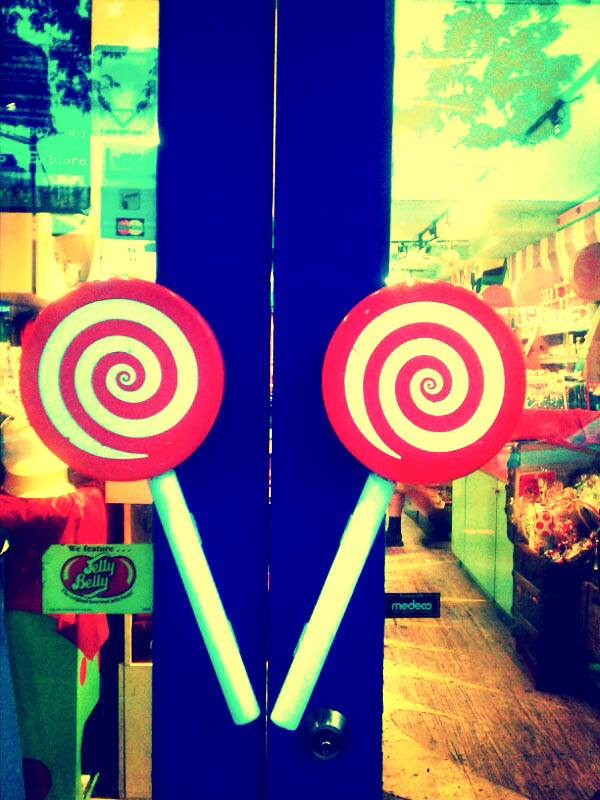The photograph showcases the entrance of a candy store with two glass double doors framed by a dark blue structure. The handles are whimsical lollipop designs featuring diagonal white sticks topped with red and white swirls. At the bottom left corner of the door, there's a white sticker advertising Jelly Belly jelly beans, displaying an image of a bean being cracked open. Above this sticker, another smaller decal indicates the acceptance of MasterCard, represented by a logo. Inside the store, although slightly obscured and blurry, colorful displays and candy assortments are visible, suggesting a vibrant and inviting atmosphere. The floor seems to be made of brown wood, contrasting with the predominantly green hues in the upper part of the image.